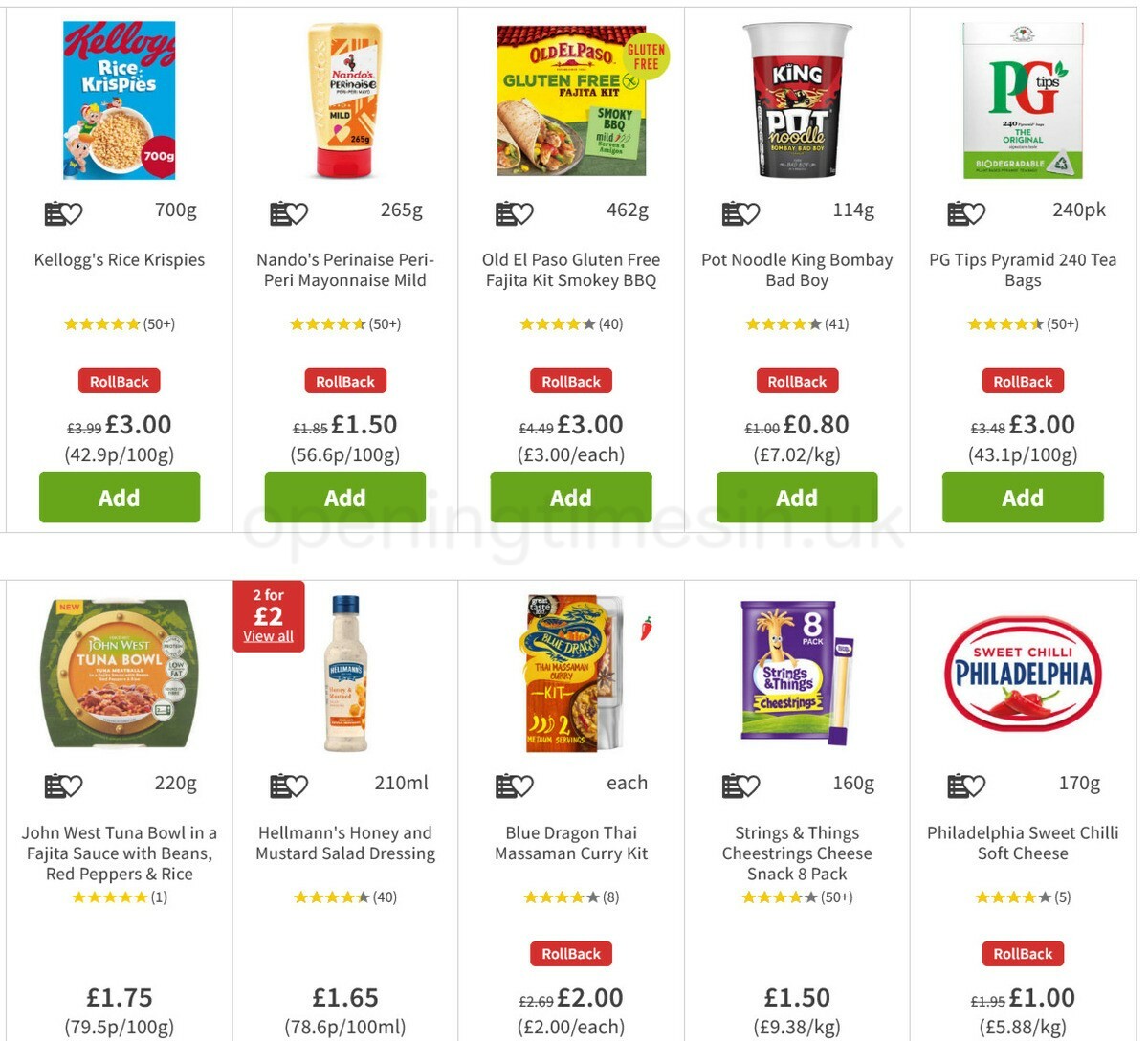The image displays a page from a grocery store advertisement featuring several items on sale. The layout consists of rectangular sections with white backgrounds and light gray borders arranged in two rows of five. Each segment is aligned side by side, touching except where a new row begins.

In the top row, the first item on the left is a blue box of Kellogg's Rice Krispies cereal, rated 5 stars with over 50 ratings. It's marked with a "Rollback" label, indicating the price was reduced from £3.99 to £3. The cost per 100 grams is listed as 42.9 pence. Beneath the price, a green "Add" button is displayed.

To the right of the cereal is a plastic squeeze tube of Nando's Perinaise Peri-Peri Mayonnaise Mild, rated 4.5 stars with over 30 ratings. It also features a "Rollback" label, showing a reduced price of £1.50.